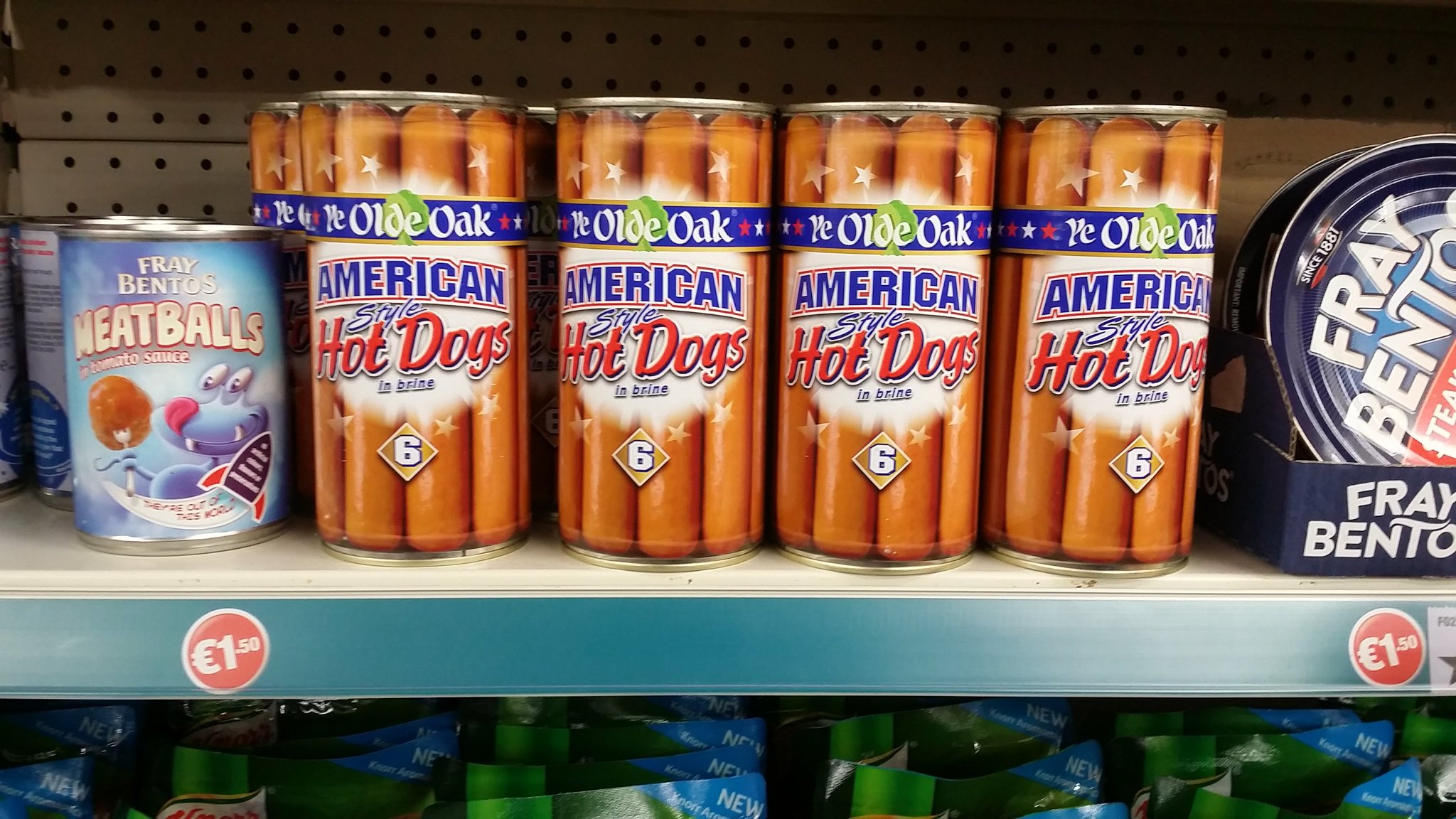The image depicts a store shelf displaying various canned goods not commonly found in American supermarkets. On the left side, there are cans labeled "Fray Bentos Meatballs." Next to these, four cans of "Old Oak American Hot Dogs," each containing six hot dogs, are lined up. The right side of the photograph is partially cut off, but it reveals the beginning of another Fray Bentos product, though the specific item remains unclear. The pricing labels on the shelf are marked with a currency symbol that is not the dollar sign, suggesting this store is located outside the United States, potentially in a European country.